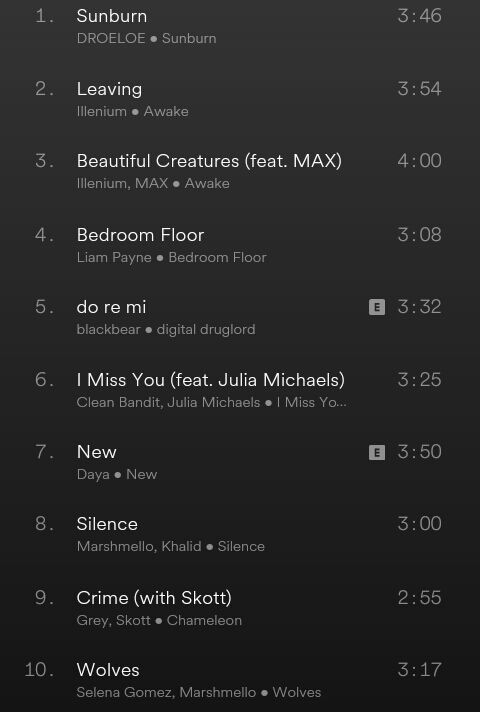Screenshot of Music Playlist from a Mobile Device

This image captures a screenshot of a music playlist, likely from a streaming service, displayed in portrait format on a mobile device such as a tablet or phone. The app does not resemble the usual interface of common platforms like Spotify. The background is a dark grey, almost black, while the text is displayed in varying shades of grey and white, providing a high-contrast, easy-to-read format.

The playlist comprises ten songs, each formatted with the track number on the left in grey, followed by the song title and artist in crisp white text. The duration of each track is noted on the right. Below are the details of the listed tracks:

1. **Sunburn** by DROELOE - 3:46 minutes
2. **Leaving** by Illenium from the album "Awake" - 3:54 minutes
3. **Beautiful Creatures** (featuring MAX) by Illenium from the album "Awake" - 4:00 minutes
4. **Bedroom Floor** by Liam Payne from the album "Bedroom Floor" - 3:08 minutes
5. **Do Re Mi** by Blackbear from the album "Digital Druglord" - 3:32 minutes
6. **I Miss You** (featuring Julia Michaels) by Clean Bandit - 3:25 minutes
7. **New** by Daya from the album "New" - 3:50 minutes
8. **Silence** by Marshmello featuring Khalid from the album "Silence" - 3:00 minutes
9. **Crime** by Grey and Skott from the album "Chameleon" - 2:55 minutes
10. **Wolves** by Selena Gomez and Marshmello from the album "Wolves" - 3:17 minutes

This detailed list provides a clear view of the song titles, artists, and durations, painting a vivid picture of the user's music preferences.